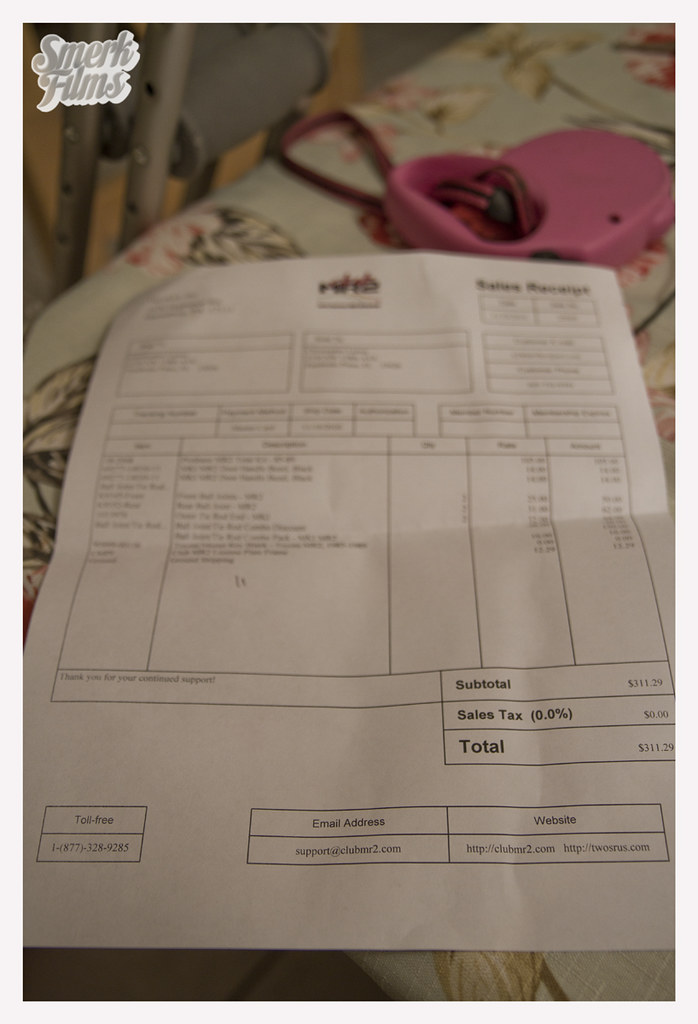An angled view looking down at a large, folded full-page receipt lays on a sage green tablecloth adorned with pink and tan floral accents. The receipt, primarily black and white, features various itemized boxes throughout. The top left corner displays a gray "MARK Films" logo against a white background. The subtotal and total at the bottom right both read $311.20, with a sales tax of 0%. Below, a box lists a toll-free number (1-877-732-8925), the email address support@clubmr2.com, and the website twosareus.com. In the top right of the image, part of a pink extendable dog leash with a plastic retractor case is visible. The scene suggests an indoor setting with a metal pole in the distant background.